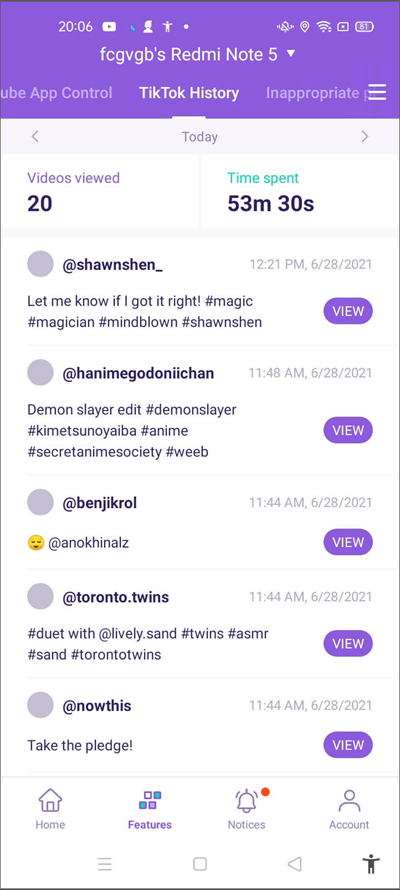A smartphone screen shows a user accessing their TikTok history. The display reveals that they have viewed 20 videos, spending a total of 53 minutes and 30 seconds on the app. Below this summary, a few timestamps of recently watched videos are listed: one at 12:21 p.m., another at 11:48 a.m., and three rapid-fire views at 11:44 a.m., indicating the shorter duration of those clips. The phone's status bar at the top of the screen shows the time as 8:06 p.m., along with a strong signal and approximately three-quarters battery life. Above the TikTok history section, a text caption reads "FCGVGBs read me note 5." On the right side of the screen, a hint of the YouTube app control can be seen, although it is not the focus. The "time spent" text is highlighted in green, and at the bottom of the screen, various notices are visible, with one marked by a red dot.